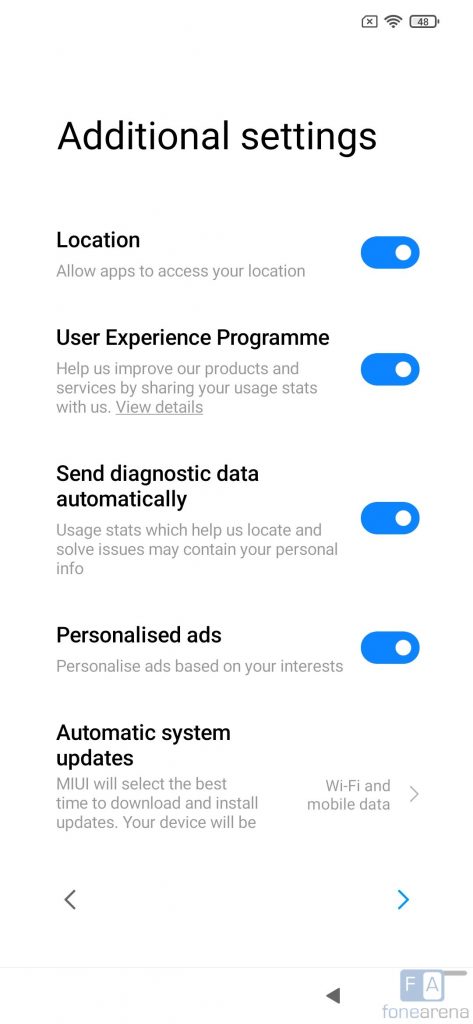This is an image of a phone's additional settings menu. At the top-right corner, the screen displays the Wi-Fi icon and a battery percentage which appears to be 40 or 48%, though the font is very small and black. Just below these icons, in black font, it says "Additional Settings."

The first option listed is "Location,” followed by the statement "Allow apps to access your location," with a blue circle containing a white dot aligned to the right.

The next line reads "User Experience Program" with a description below: "Help us improve our products and services by sharing your usage stats with us." Next to this text, there's a blue circle with a white dot on the right, and an underscore labeled "View details."

Following this is the option "Send diagnostic data automatically," which explains: "Usage stats which help us locate and solve issues may contain your personal info." Again, a blue circle with a white dot is positioned to the right.

The next option is "Personalized ads," offering "Personalized ads based on your interests," with the same blue circle and white dot to the right.

Then, we have "Automatic system updates," stating that "MIUI will select the best time to download and install updates." To the right, it specifies "Wi-Fi and mobile data" with a gray arrow pointing to the right.

Further down, there’s some additional navigation: a gray arrow to the left, a blue arrow to the right, and a gray line. To the right side, there is a black triangle pointing left. Below that, in a blue box with white lettering, it says "F" and in a white box with black lettering, it says "A." Below these, in gray text, it reads "fonearena."